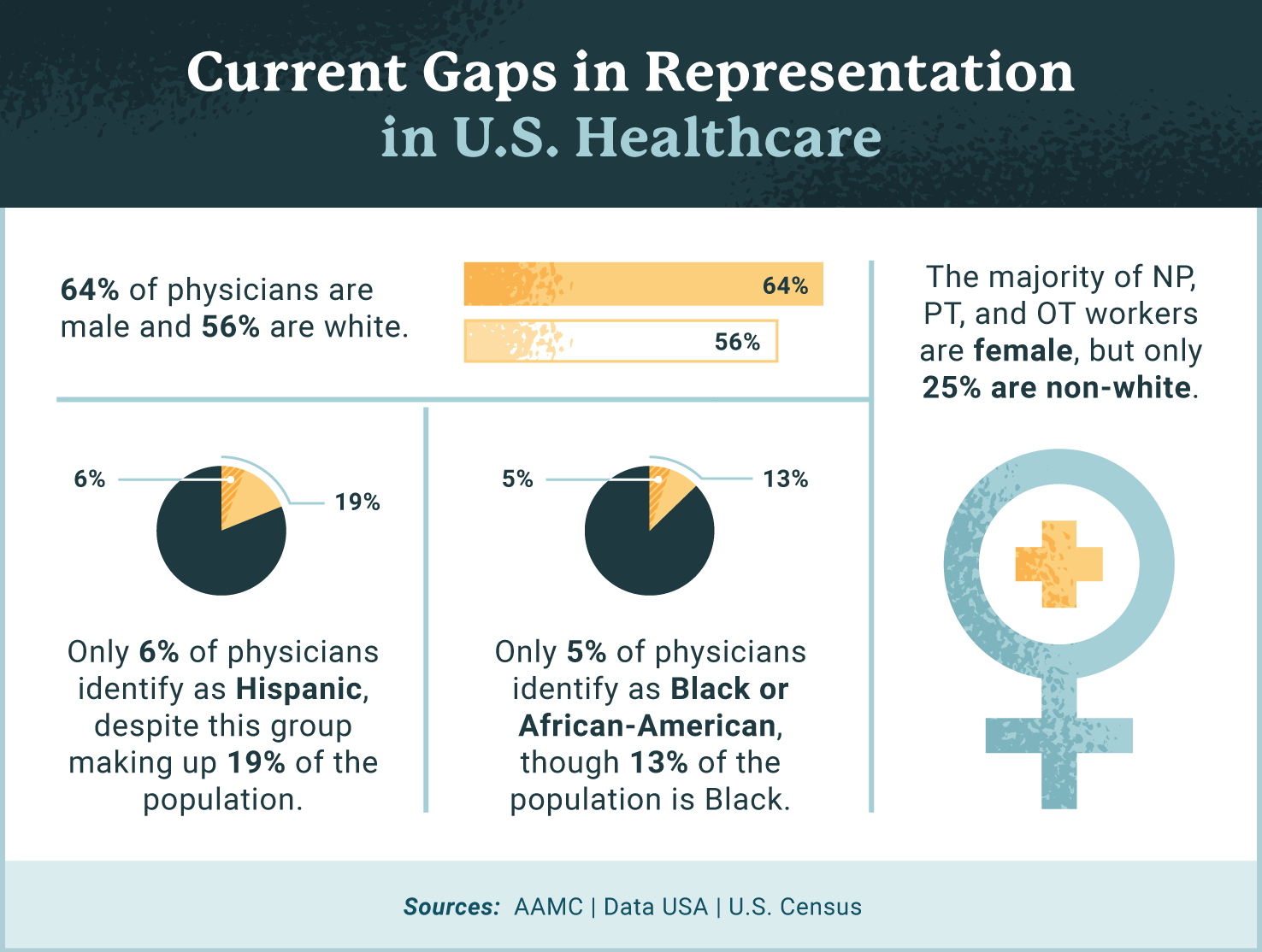The image is a color infographic in a landscape orientation designed to present current gaps in representation within U.S. healthcare. At the top, a black horizontal strip features white text reading "Current Gaps in Representation," with blue text underneath stating "In U.S. Healthcare." Below this, against a white background, different sections highlight key statistics through bar graphs and pie charts. 

On the left, an orange bar graph indicates that 64% of physicians are male, while an orangish-white bar graph shows that 56% of physicians are white. To the right, there is a section marked with the blue universal symbol for female, featuring a gold cross inside the circle, accompanied by text that reads, "The Majority of NP, PT, and OT workers are female, but only 25% are non-white."

Further to the left, two pie charts provide additional demographic details. One chart indicates that only 6% of physicians identify as Hispanic, despite Hispanics making up 19% of the population. The other chart reveals that only 5% of physicians identify as Black or African American, though 13% of the population falls into this demographic. 

At the bottom of the infographic, a blue horizontal band contains the sources for this data: AAMC, DataUSA, and U.S. Census.